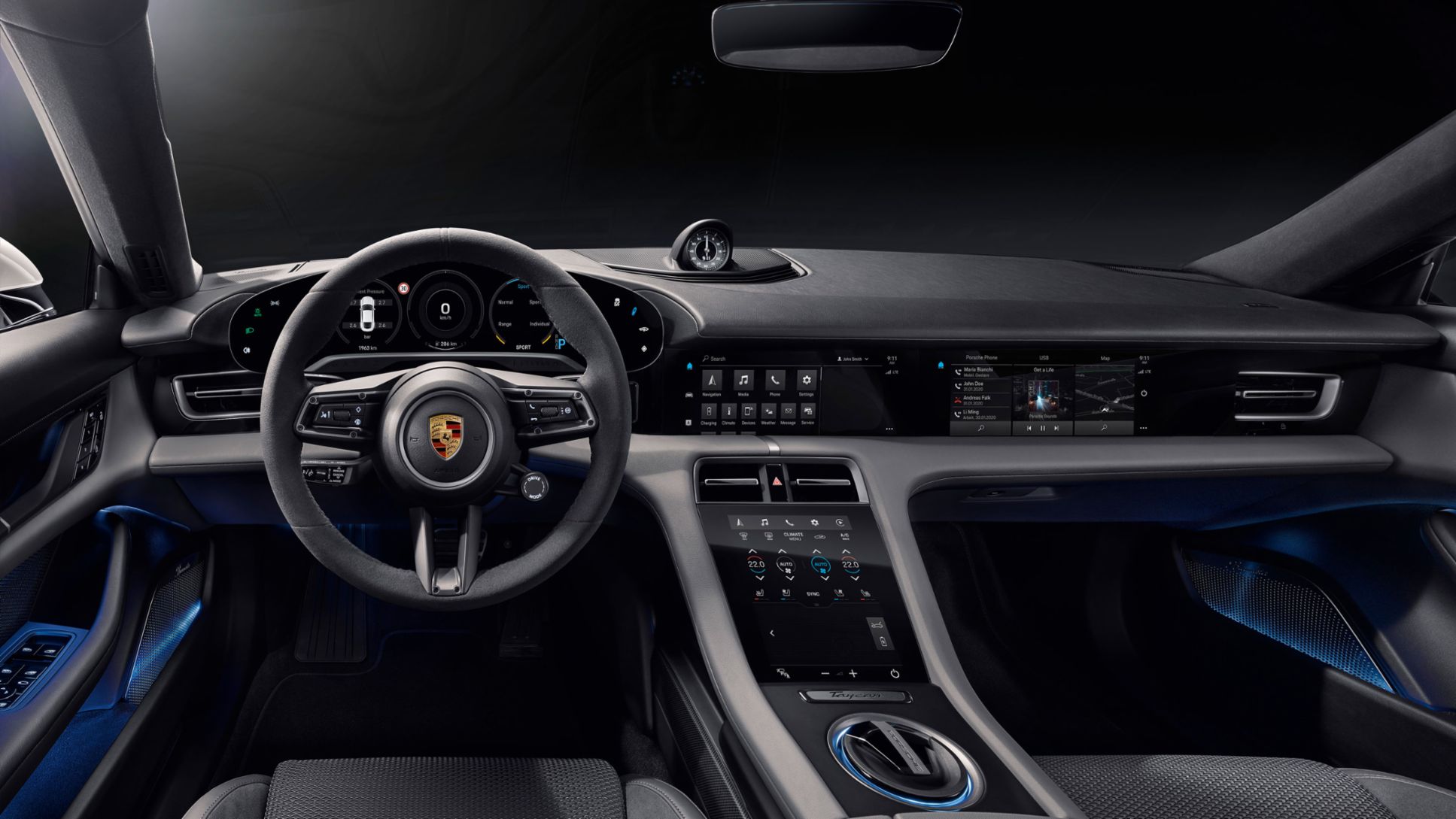The photograph, possibly AI-generated, presents a sleek and professional view from the driver's seat of a luxurious sports car, likely a Porsche, as suggested by the logo on the steering wheel. The driver's seat is located on the left side, encapsulating an ambiance of modern sophistication with its predominantly black interior accented by various shades of gray. Soft blue under-head lights glow subtly on the door panels, illuminating the handles and adding a touch of futuristic elegance. A meticulously designed dashboard features a central clock, contributing to the car's refined aesthetic. The front windshield appears to be covered, creating a pitch-black backdrop that draws attention to the illuminated and stylishly designed interior. A cup holder is conveniently positioned in the middle, complementing the car's functional yet polished design.